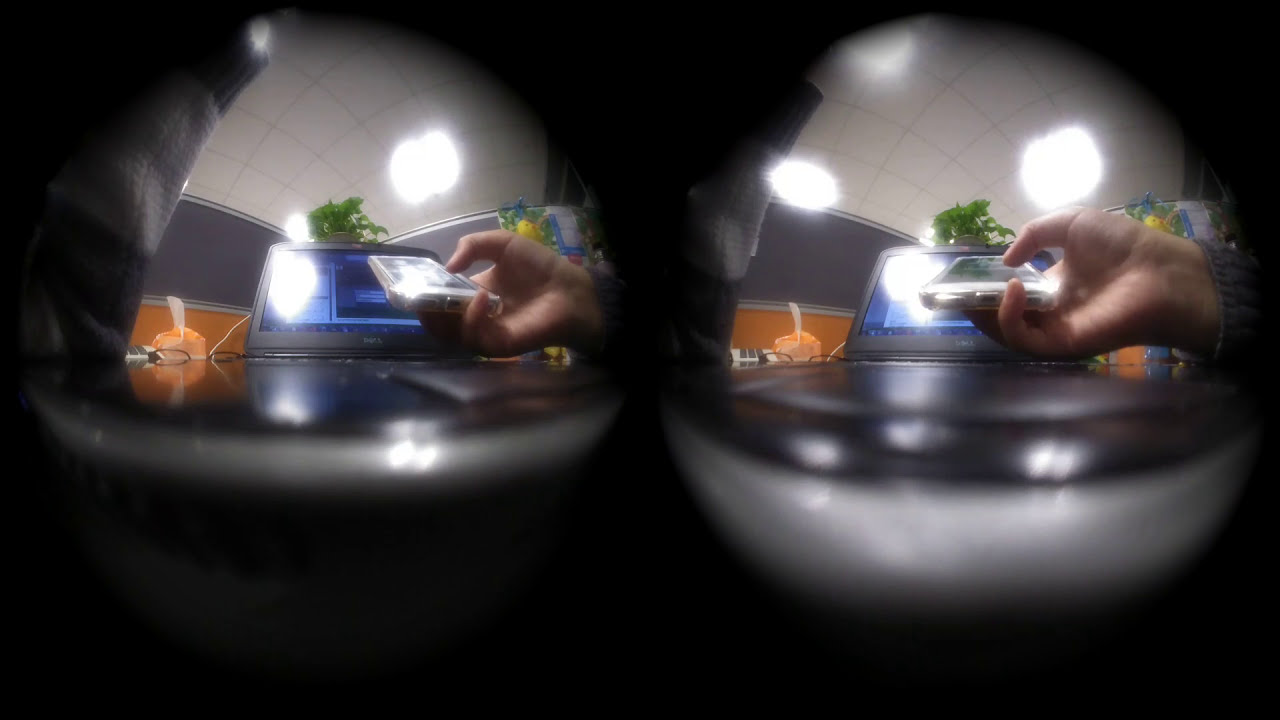The image depicts a blurred and slightly distorted scene captured through a dual, oval viewing window, possibly resembling keyholes or eye-like shapes. The photograph has a black surrounding border and appears to exhibit a double exposure of the same shot, with one frame slightly zoomed in or tilted compared to the other. At the center, a right hand is gripping a cell phone, likely an iPhone, with a minimal view of its sleeve, poised against a black Windows or Dell laptop in the background. Bright white lights from a grid-marked ceiling cast a reflective glow onto the phone and laptop screens. Behind the person's hand and phone, the setting appears to be an office desk, featuring a dark blackboard or wall and an orange lower wall, along with a small, indistinct digital device. Additional elements include an orange bag or item and perhaps a tissue box near the laptop. The photograph has an overall surveillance-like quality, emphasizing the ambient office environment with its distinct furnishings and lighting.